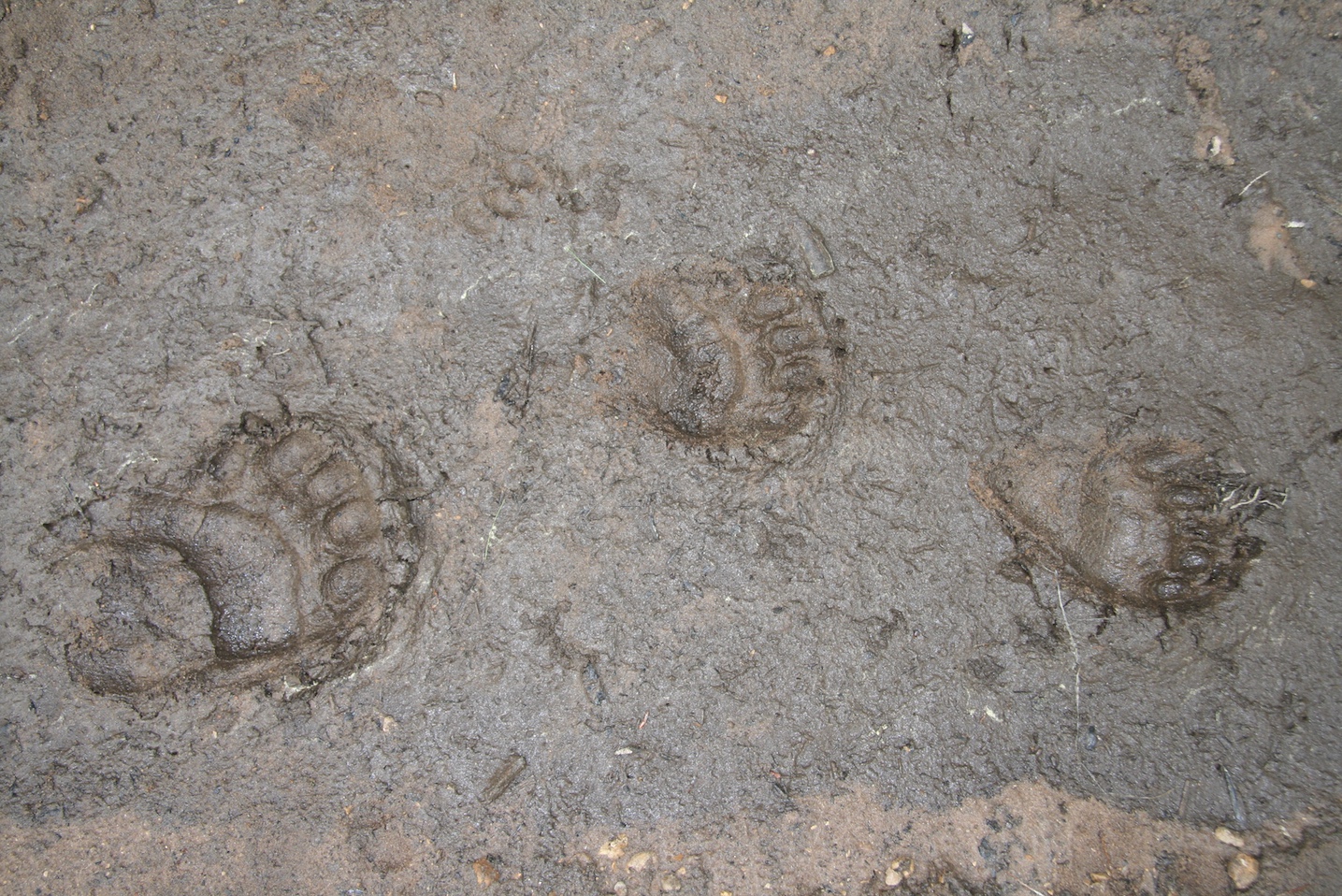This image captures a textured expanse of dirt or wet sand, characterized by a gritty and crackled surface indicative of a drying environment. Scattered small pebbles dot the scene, especially concentrated towards the edges. Featured prominently are three distinct sets of footprints. On the left side, a significantly larger animal footprint is clearly visible, its size and markings suggesting the presence of a substantial creature. In the center, a much smaller footprint, approximately half the size of the larger one, is imprinted into the sand. To the right, an obscure and less detailed third footprint appears, differing from the other two in shape and clarity. The variety in footprint sizes and shapes hints at the passage of different animals across this landscape, adding a narrative element to the gritty, time-worn surface.